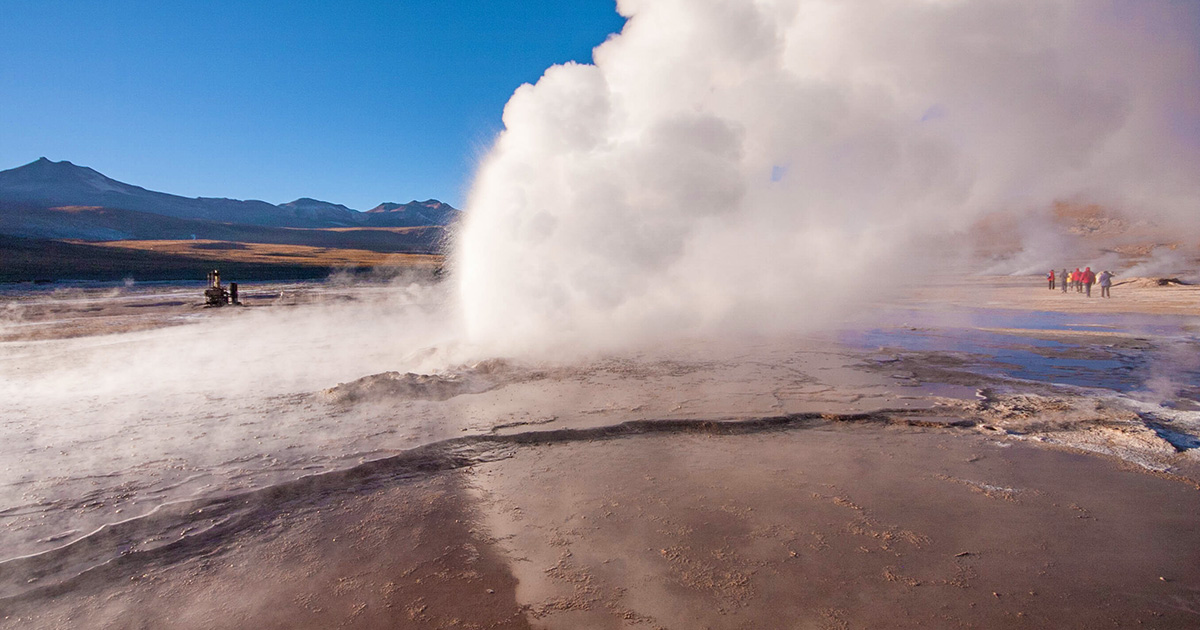The photograph captures a mesmerizing scene at a geothermal field, likely resembling the famous El Tatio located in the Andes Mountains of northern Chile. The image foreground displays a muddy, reflective terrain with a brown and beige hue, interspersed with numerous billowing clouds of steam. At the center, a substantial plume of mostly white, accented with gray smoke, rises dramatically above a possible geyser or geothermal vent. This plume bends toward the right side of the photograph, where a group of tourists can be seen. These individuals, appearing small in the distance, are distinguishable by their colorful jackets: three in red, one in yellow, two in gray, and one in purple. The backdrop features a clear, cyan blue sky streaked with white near the horizon, behind a jagged mountain range. The time of day appears to be midday, as suggested by the brightness of the natural light. Overall, the scene exudes a rugged, yet serene, natural beauty, underscoring the geothermal wonders amidst a tranquil Andean landscape.